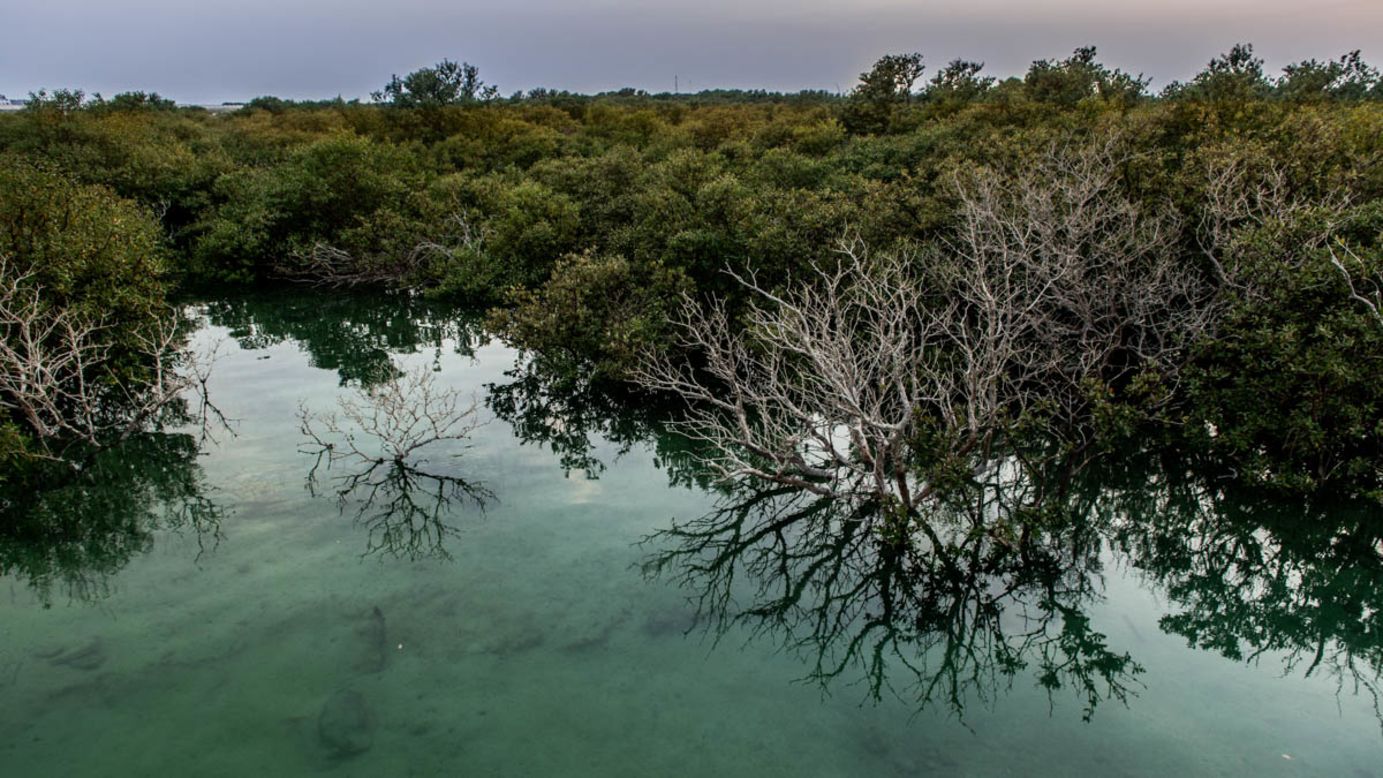This vivid outdoor photograph appears to capture a scene reminiscent of the Florida Everglades or a similarly swampy area, possibly even a dense rainforest. The foreground is dominated by a pond or lake with murky, dark blue water that almost resembles quicksand or sludge at the bottom. The water is interspersed with both living and dead trees, some with whitish gray, leafless branches, whose reflections can be seen rippling on the water's surface. Surrounding the water is a lush landscape of thick green bushes and shrubs, creating a dense, vibrant forest. The background features a tree line that stretches far into the distance, adding depth to the image. Above all this, the sky is overcast with grayish purple clouds, contributing to the moody, somber atmosphere of the photograph.